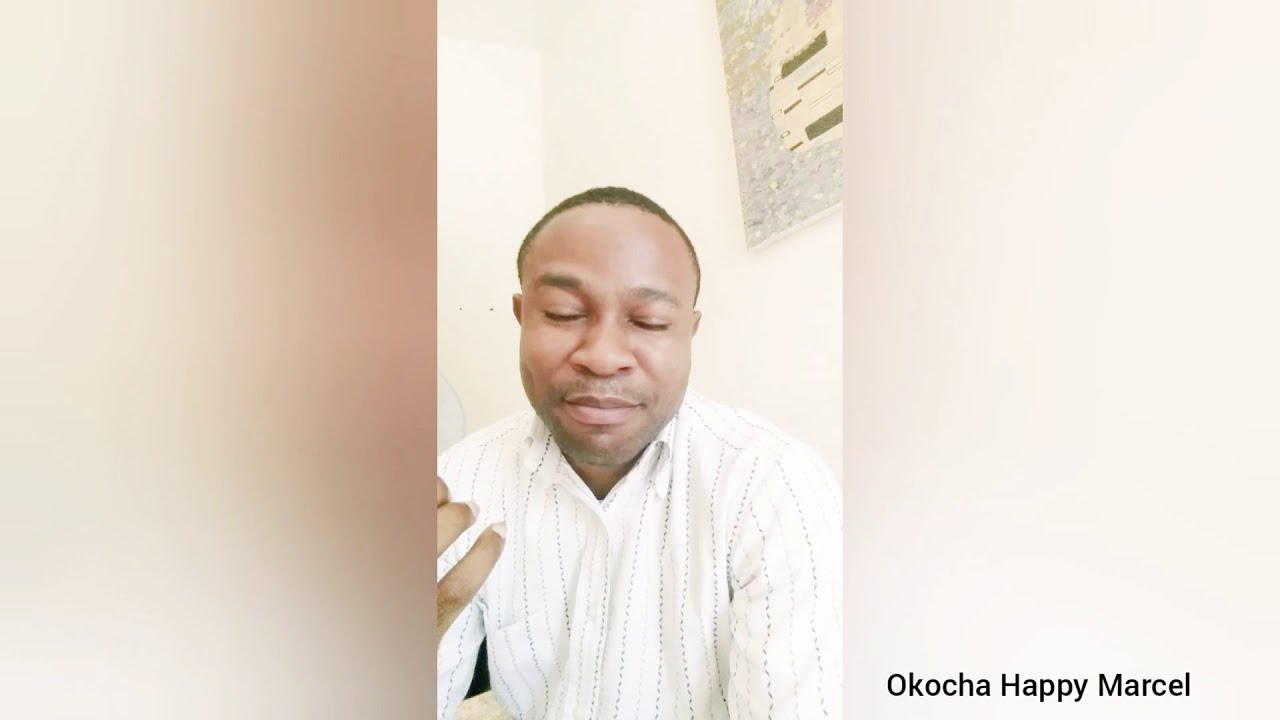The image appears to be a still from a TikTok or cell phone video, depicting an African-American man from the stomach up. He has short black hair and a stubbly beard, with his eyes closed and his mouth mid-sentence, suggesting he might be speaking or emphasizing a point. He is dressed in a long-sleeved, white button-down shirt adorned with black striped dots. His right hand is raised, with the tips of his fingers slightly curled inward. The background features a plain white wall, with a decorative piece of art visible in the upper right corner—a canvas with a gray background and a light tan and green design. Light tan borders flank the image on both sides. In the bottom right corner, black text reads "Okocha Happy Marcel."